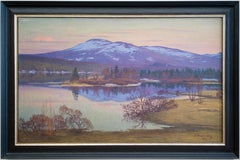The image is a small, framed landscape painting depicting a serene lakeside scene. The black frame with a gold inner border encloses a vibrant portrayal of nature. In the foreground, there is a grassy field leading up to the edge of a lake. A few trees are scattered along the shore. The lake itself is calm and highly reflective, mirroring the scenery around it. In the center of the lake, a grassy island with a few trees stands serenely. The far bank of the lake features a juxtaposition of a large wooded area to the right and a tall grassy field to the left, both leading the eye to a majestic, snow-capped peak in the distance. Above the peak, the sky is mostly blue with some clouds, adding to the sense of depth and tranquility. The reflection of the snowy peak and surrounding trees in the lake's pristine waters enhances the natural beauty of the scene, while hints of fall colors in the trees and slight haze in the sky imbue the painting with a seasonal charm, possibly indicating an autumn morning.